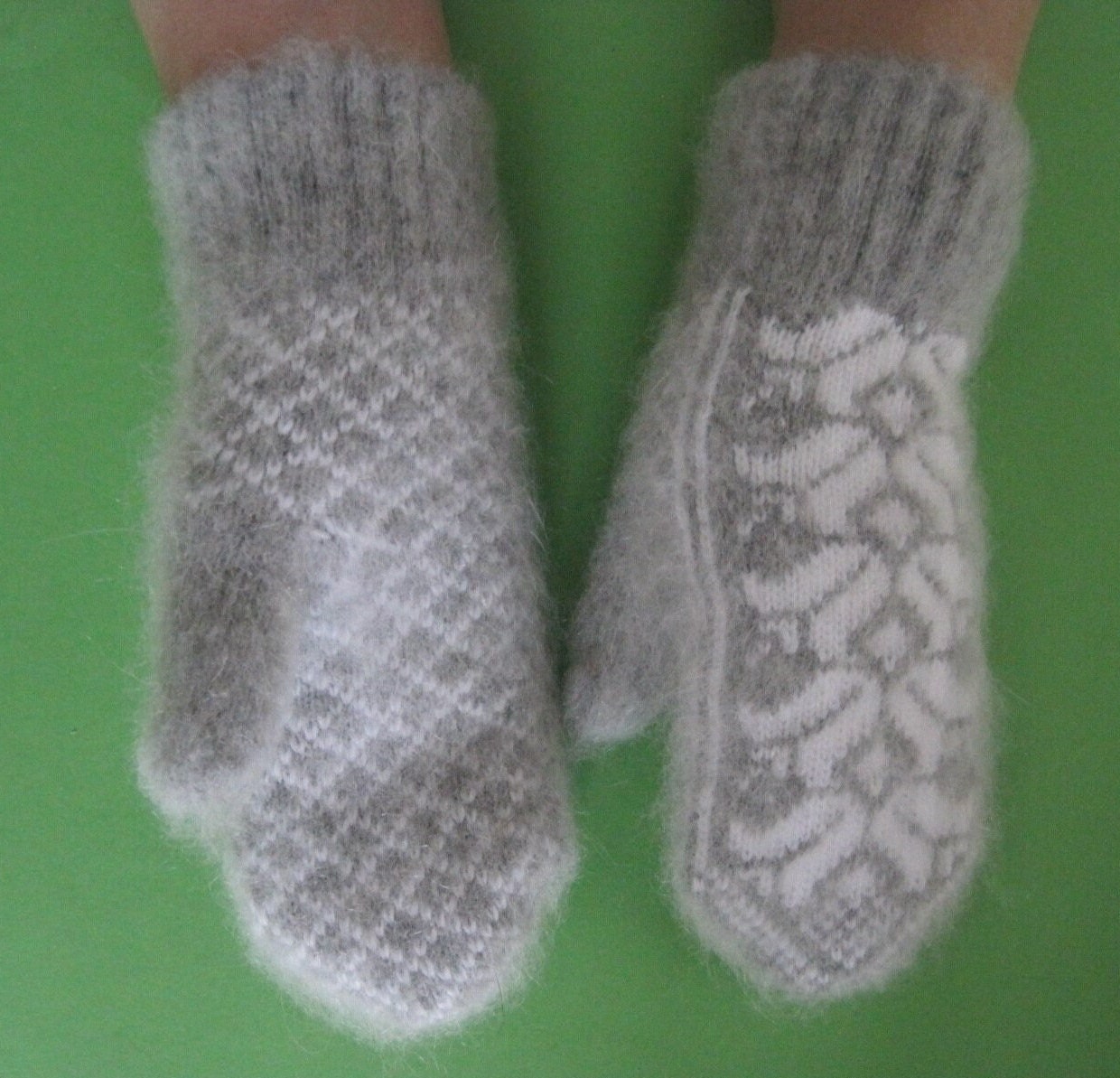This is a color photograph taken indoors, featuring a green fabric backdrop. At the top of the image, there are two hands adorned in wool knit mittens, exhibiting a noticeable degree of fuzziness from the fibers. The arms are slightly visible at the top right and top left. The left hand, positioned with the palm facing up, displays a light gray mitten decorated with a white crisscross pattern. In contrast, the right hand is shown with the palm facing down, revealing the back of the mitten adorned with an intricate white pattern that includes floral or leaf designs with diamond centers, extending from the wrist to the fingertips. The mittens provide a detailed, cozy texture, highlighting the craftsmanship and pattern work.